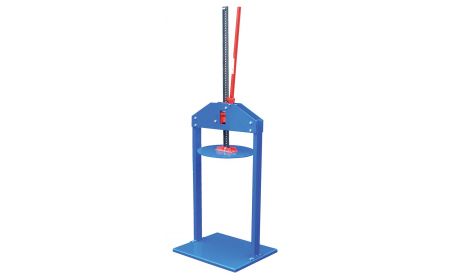The image depicts a small, mechanical device with a simple design set against a completely white background, giving it a transparent and clean look. Its orientation is portrait, and it appears to be almost thumbnail-sized. The structure consists predominantly of blue, red, and silver colors.

The base of the device is a metallic blue square, from which two blue metallic vertical posts rise. These posts are positioned on opposite sides of the base, extending upward. At the top, the posts are connected by a rectangular blue bracket. Through this bracket runs a central silver metal rod, which seems to be threaded. Attached to the rod is a red metal component that extends downward, passing through the bracket and reaching towards a circular, blue disc situated below the bracket, in the mid-section, supported by the uprights.

The functional purpose of this device is ambiguous. The red piece moves along the threaded rod, suggesting it could act as a press or vice mechanism, possibly for compressing or holding objects. The circular disc at the bottom might serve as a supporting or moving part of this function. Despite the detailed structure, the exact use of the device remains unclear, as there are no additional texts or hints to clarify its purpose.